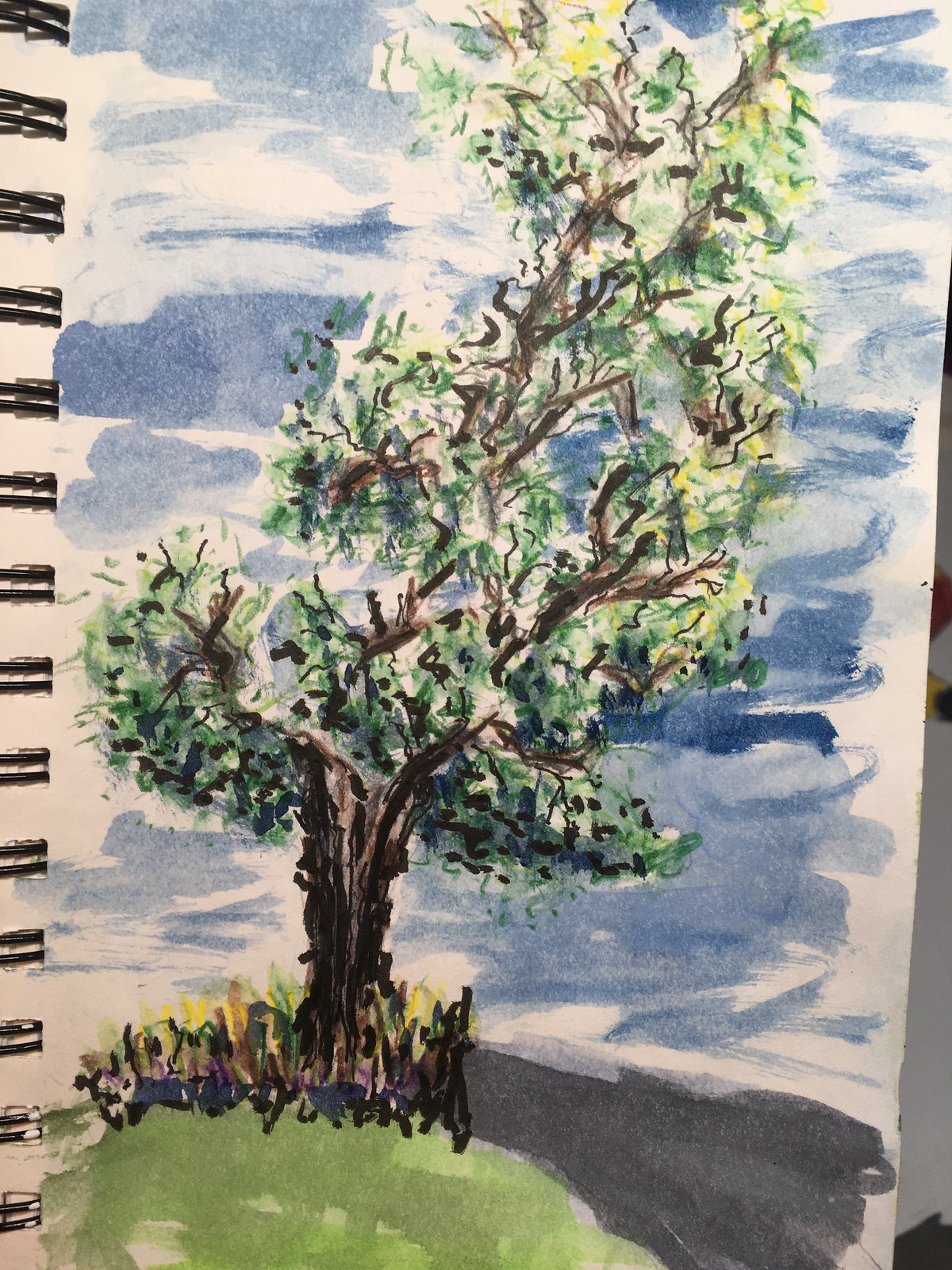The image depicts a detailed watercolor sketch on a ring-bound, vertical rectangular sketchbook with thick, cottony-feel paper. The dominant feature is a tree with a brown trunk, slightly leaning to the right, surrounded by tall branches adorned with green leaves and small yellow flowers or berries. Below the tree, there is a mound of murky green grass interspersed with lighter patches, giving the illusion of light hitting it. Surrounding the base of the tree are rough brown and green squiggles representing weeds and other undergrowth. Most of the sky, painted with blue daubs, occupies the upper three-quarters of the page, providing a backdrop to the scene. To the left of the sketch, the black spirals of the notebook are visible, holding the pages together. The overall presentation has a scrappy, rough charm, characteristic of a casual yet expressive watercolor artwork.